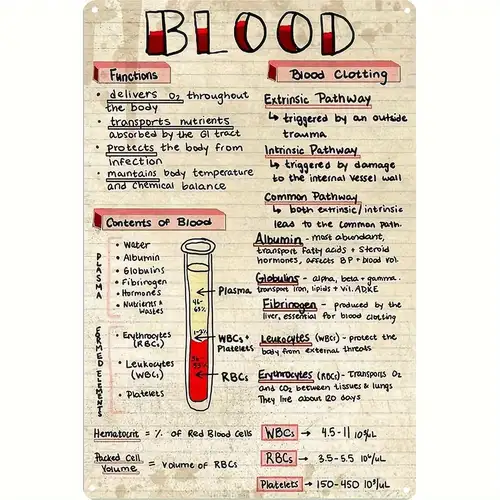This image shows a neatly written and detailed notebook page in a tan color, evidently taken from a biology or scientific lecture. At the top, the word "Blood" is prominently displayed in bold block lettering, with the left half of each letter filled in bright red, symbolizing blood. Key sections are boxed in red for emphasis.

On the left, under a red box labeled "Functions," there is a list detailing blood's roles: delivering O2 throughout the body, transporting nutrients absorbed by the GI tract, protecting against infection, maintaining body temperature, and ensuring chemical balance.

Mid-page, another red box titled "Contents of Blood" outlines the components of blood. It includes a subsection for "Plasma" listing water, albumin, globulins, fibrinogen, hormones, and nutrient values. Below, the "Formed Elements" subsection notes erythrocytes (RBCs), leukocytes (WBCs), and platelets.

A drawing of a vial illustrates blood composition: the red bottom portion marked as RBCs, a yellow top portion labeled plasma, and a small middle portion identified as WBCs.

Definitions and explanations continue beneath, including terms like hematocrit (percentage of red blood cells) and packed cell volume (volume of RBCs). The right-hand side features another red box titled "Blood Clotting," with a list explaining pathways: the extrinsic pathway triggered by external trauma, the intrinsic pathway triggered by internal vessel wall damage, and the common pathway merging both.

Additional notes covered include albumin's role in affecting blood pressure and volume, globulins involved in transporting iron and vitamins, fibrinogen's crucial part in clotting, and erythrocytes' CO2 and O2 transport between tissues and lungs, noting their lifespan of about 120 days.